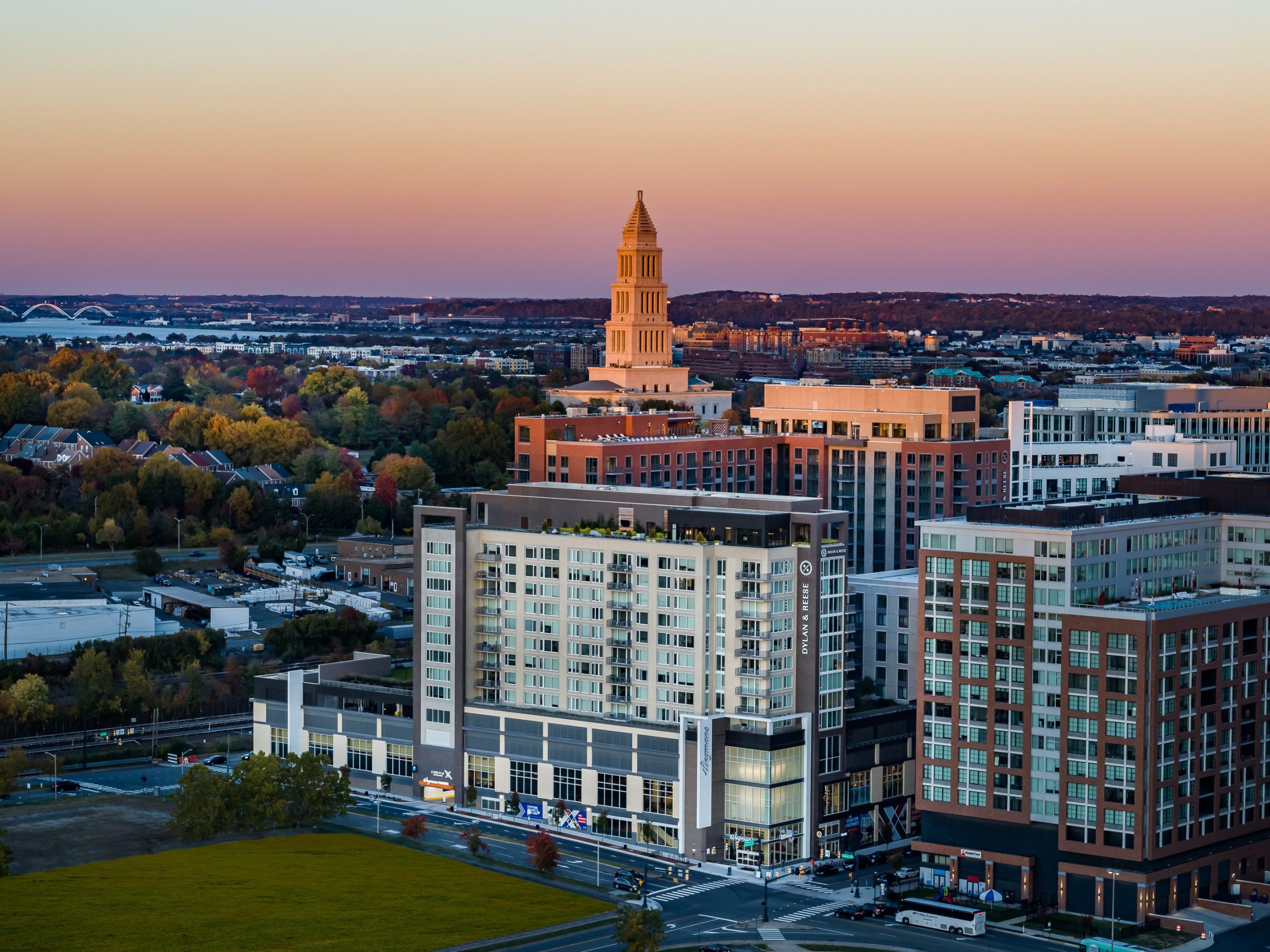This detailed aerial photograph captures a bustling modern cityscape with a diverse range of architectural and natural elements. Dominating the scene is a tall, four-level white skyscraper that tapers to a point, standing prominently among numerous other buildings of varying heights. Toward the bottom right and middle portion of the image, several multi-level apartment buildings in shades of brown, white, and gray are visible, distinguished by their numerous windows. To the left of these residential structures, a cluster of trees displays a brilliant array of fall colors, including red, yellow, and green, seamlessly blending into the nearby green space which could be a park or open field. Further left, there's a bridge near the city's edge. The foreground reveals elements of urban life, such as a parking lot and cars and buses on the roads, while the top of the image showcases hints of a mountain range in the distance and water bodies, either a small river or lake, adding to the natural beauty that intersperses this vibrant urban area. The overall scene is bathed in a warm, golden light, suggesting the photograph was taken at either sunrise or sunset.